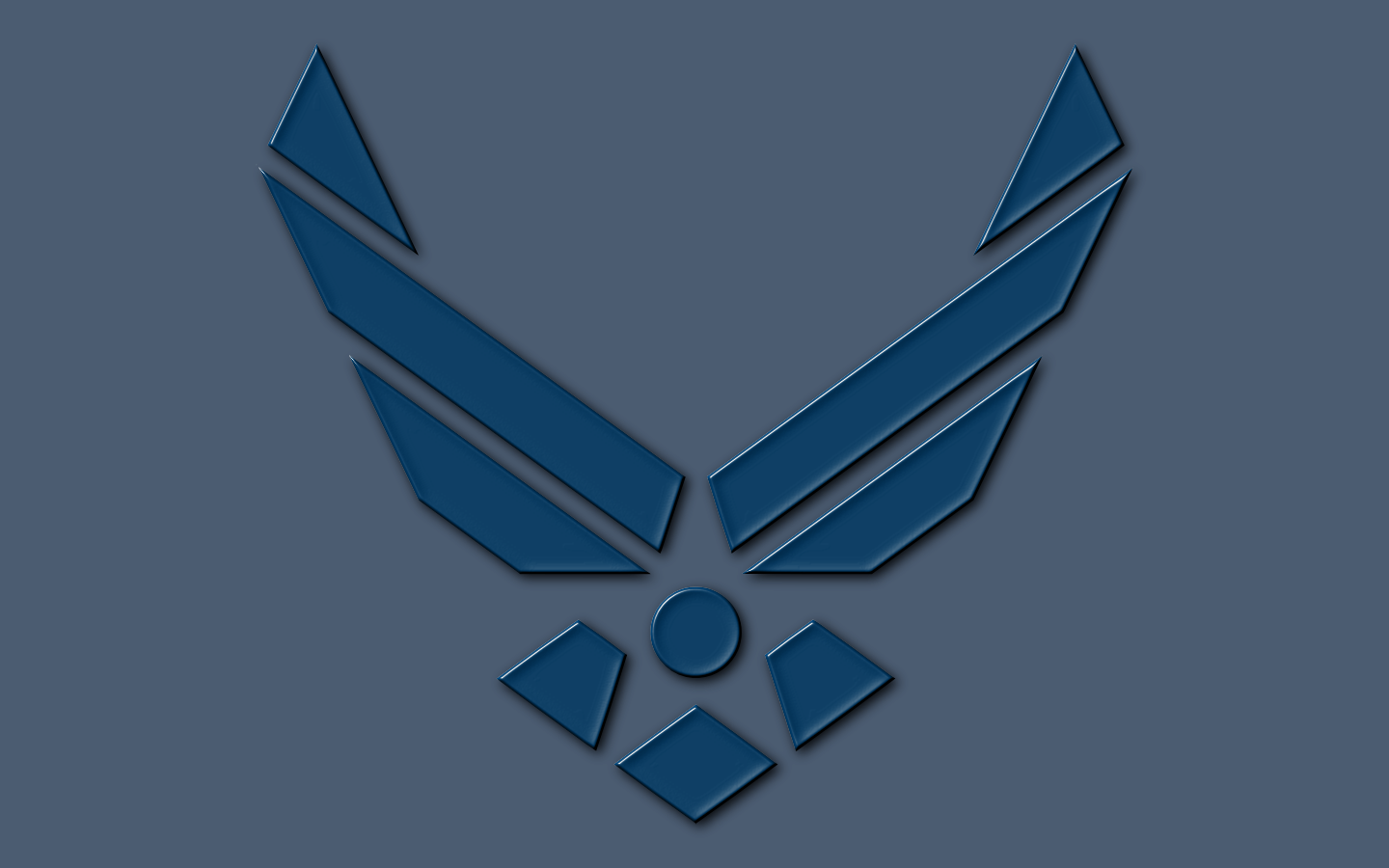The image is a horizontally-oriented graphic, featuring a high-tech logo on a dull, bluish-gray background. Dominating the composition is an embossed, symmetrical arrangement of geometric shapes in a deeper, muted blue, similar to the background. Positioned at the center of the logo is a circle, which serves as a focal point.

Above this central circle, two long quadrilateral shapes extend upwards like wings, each topped with triangles that point inwards. Directly beneath the central circle are additional geometric elements, including both large and small trapezoids, a horizontally positioned diamond, and other shapes like pentagons and longer rectangles, all maintaining vertical symmetry.

The bottom-most section includes three distinct shapes resembling diamonds or truncated pyramids, adding complexity to the overall design. The right side of the image features subtle white stripes emanating from the upper left, suggesting a light source casting a gentle shine across the logo, enhancing its high-tech appearance.

There is no text present in the image, emphasizing the logo's intricate and symmetrical design, possibly representing a modern company's insignia or a machine emblem.